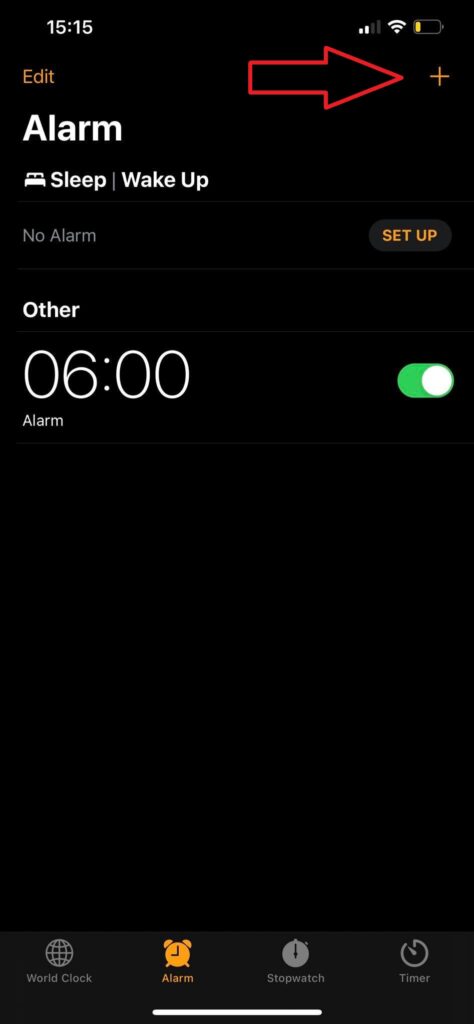This screenshot captures the alarm-setting interface on an iPhone. The clock in the top-left corner displays "15:15" in white text, accompanied by indicators showing two bars of service signal strength, active Wi-Fi, and a battery level at around 20%. 

On the left-hand side of the screen, an "Edit" option is displayed in an orangish color, situated above an alarm label that reads "Sleep | Wake Up" and features a small bed icon. Directly below, it states "No Alarm," with a corresponding "Set Up" option in the same orangish color on the right-hand side.

Further down on the left, under the "No Alarm" notification, is another section labeled "Other," with a time set to "06:00" (6:00 AM). This section indicates an active alarm, as evidenced by the toggle button switched to the right and displaying green to signify that the alarm is enabled.

A large red arrow is superimposed near the top, pointing right toward a plus sign, likely indicating where to add a new alarm.

At the very bottom of the screenshot, the screen is segmented into different features: "World Clock," "Alarm" (highlighted in the orangish-yellow color), "Stopwatch," and "Timer," which are standard functionalities within the iPhone's clock app.